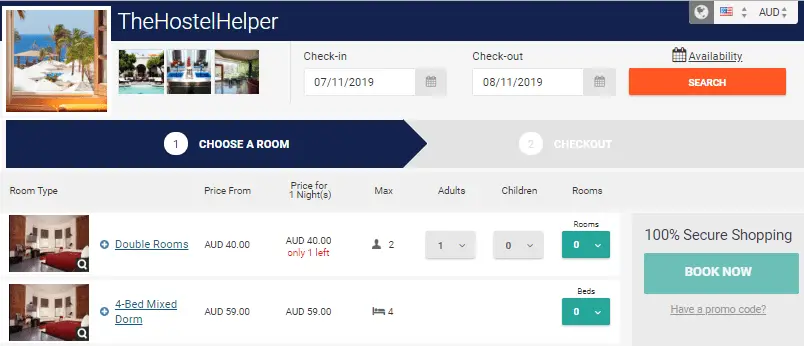In the upper left corner of the interface, there's a square image depicting a serene beach scene with the ocean, palm trees, sun loungers, and a brown hut or canopy area. To the left of this image, in white text, is written "The Hostile Helper," alongside the check-in date of "7-11-2019" and the check-out date of "8-11-2019." Adjacent to this, an orange rectangle features the word "Search."

Below, the interface offers booking options with two tabs: "Choose a Room" against a blue background marked as option one, and "Check Out" against a gray background marked as option two. The room types are listed with details: 

1. A double room priced from AUD $40 per night, accommodating a maximum of two adults, currently showing availability of zero rooms. 
2. An image of the double room is displayed with a red bed and windows. 

Beside this image, details for a four-bed mixed dorm are provided, citing a price of AUD $59 per night and accommodating up to four individuals. A green box underneath indicates the number of beds available (currently zero), with an arrow for adjusting this number according to the guest's needs.